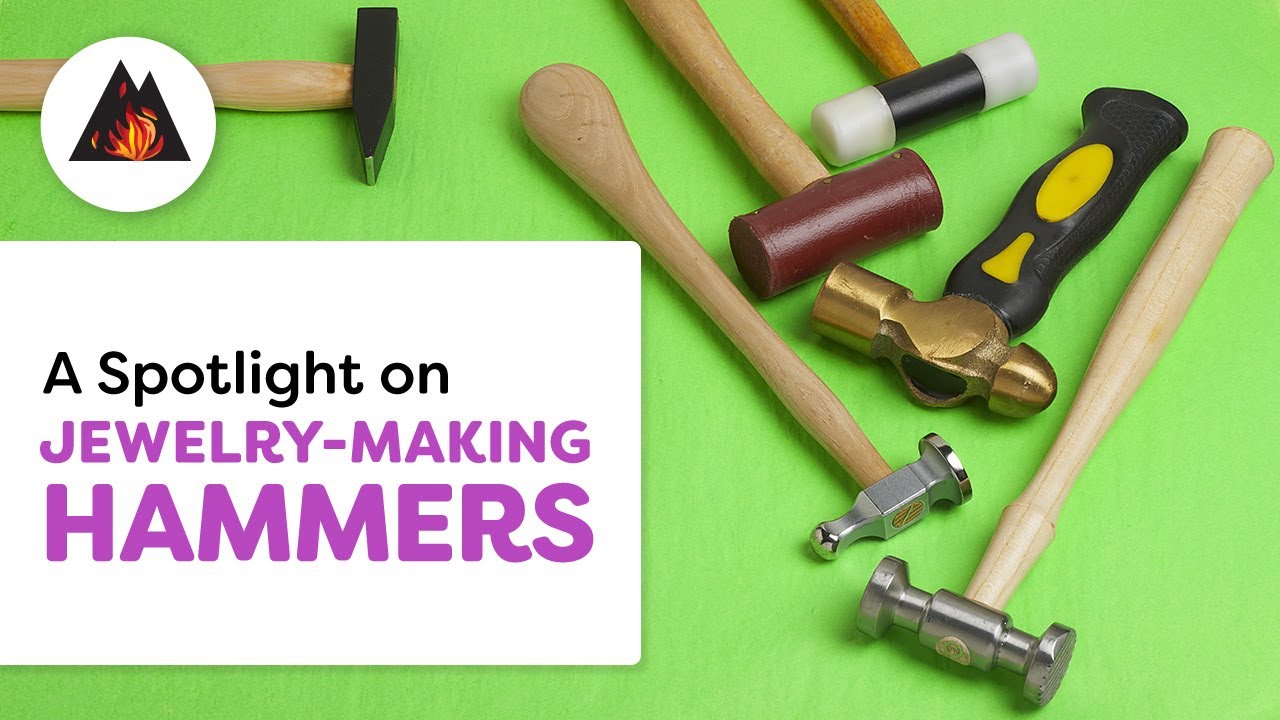This image features an advertisement titled "A SPOTLIGHT ON JEWELRY MAKING HAMMERS." The title is displayed within a white rectangle on the left side, with "spotlight on" in black text and "jewelry making hammers" in bold purple capital letters. Above this text box, a logo is also visible. The background showcases six distinct hammers neatly arranged on a green surface, each designed for specialized tasks in jewelry making. The hammers vary in head shapes and colors, including silver, bronzy gold, maroon, and black. Notably, one hammer has a black handle with two yellow shapes, while the rest feature natural wooden handles. Another hammer has a dual-colored head with white ends and a black center. This detailed layout emphasizes the unique qualities and diversity of tools essential for the intricate craft of jewelry making.